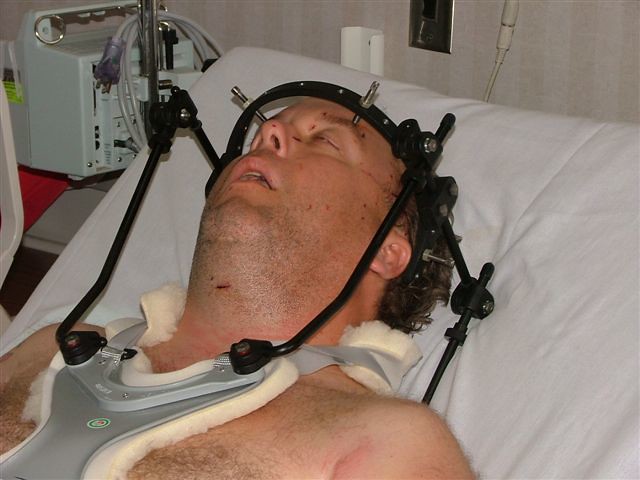The close-up image shows a man lying in a hospital bed, appearing unconscious or asleep, with his eyes mostly closed and mouth slightly open. He is wearing a black medical halo device around his head, secured with screws into his forehead, which extends down to a silver vest covering his collarbone. The vest features a padded tan lining and white foam underneath for cushioning. The man, who has a slightly hairy chest and stubble on his chin, is not wearing a shirt. Surrounding him is a sparse hospital environment: a small piece of machinery is visible to the upper left of the image, and a tan striped wall forms the background behind the white hospital bed sheets.